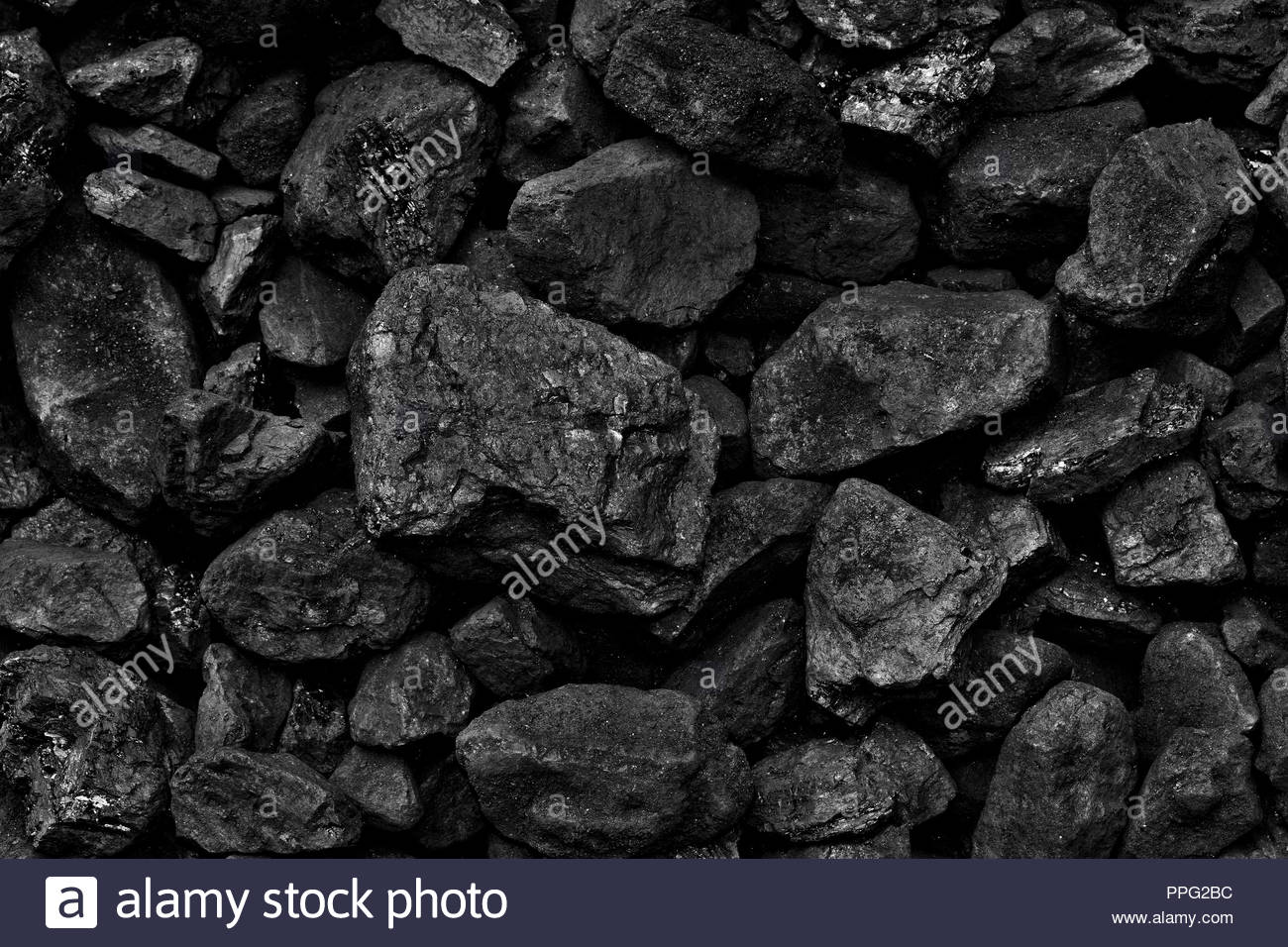This close-up stock photograph, possibly in black and white due to its overall dark tones, showcases a large mass of coal or dark granite-like rocks. The image is vertically rectangular, filled with variously sized and shaped stones or coal chunks, all fitting within the palm of a hand. The rocks range in texture from glistening to dull, with some having shiny flecks. Diagonal rows faintly spell out "A-L-A-M-Y," which appears throughout the image as a trademark assurance. At the bottom, a dark purple strip with white text reads "Alamy stock photo," featuring an "A" in a square logo, and accompanying the logo is a smaller text on the right, "PPG 2BC www.alamy.com," likely referencing the image’s catalog information.